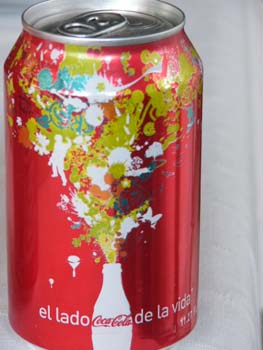This image features a vibrant red aluminum can of Coca-Cola with a polished, silver top where the can opener mechanism is clearly visible. This opener, when lifted, pierces the seal to create a mouthpiece to drink from. The central design element of the can is particularly eye-catching: it depicts a stylized bottle that appears to be bursting open, releasing an artistic cascade of people, butterflies, and paint splashes. This dynamic composition lends the can a very cool and creative vibe. At the bottom of the can, the text "Helado Coca-Cola de la Vida" is prominently displayed, indicating that the design and possibly the flavor are themed around a refreshing and lively concept, adding an international touch with its Spanish phrasing.